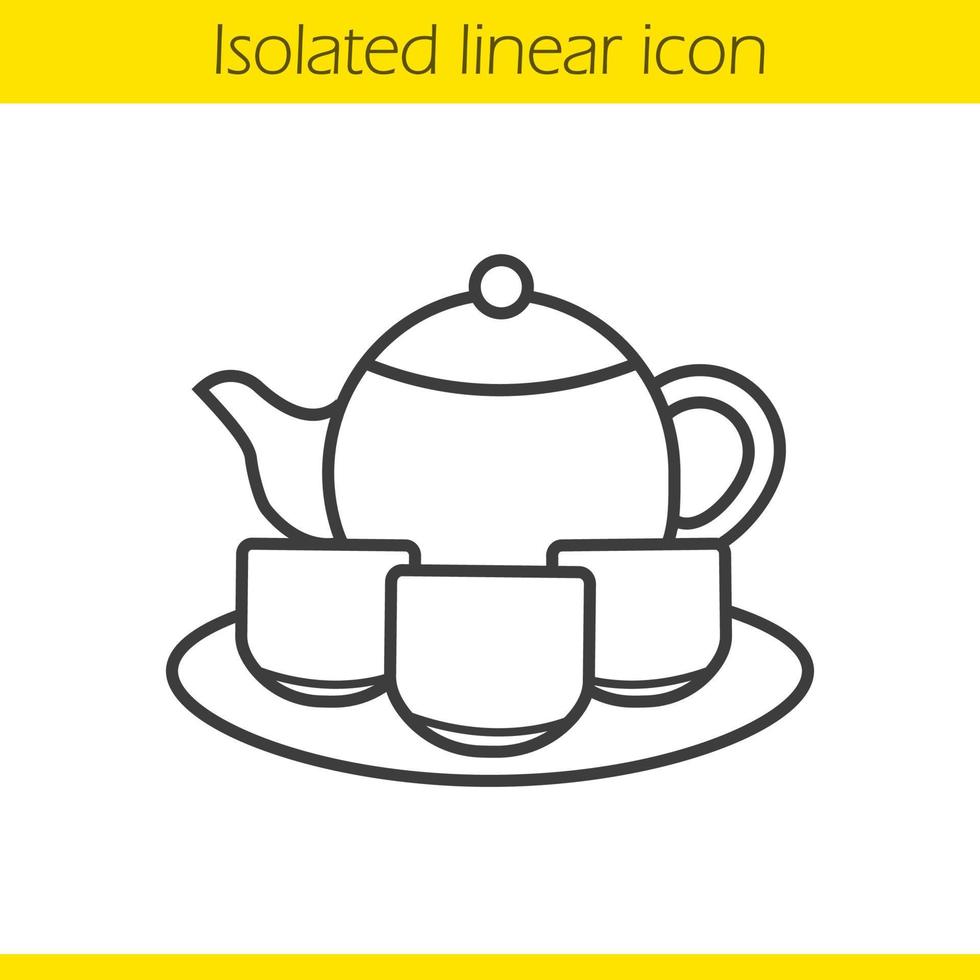The image is a black-and-white sketch with minimal details, highlighted by two vivid yellow banners. The prominent yellow banner at the top stretches across the entire width and features the text "Isolated Linear Icon" in bold black letters. Below the image, a thinner yellow ribbon extends from left to right without any text. The central illustration depicts a round teapot with a small handle on the right side and a spout on the left. It has a lid with a knob for lifting. Accompanying the teapot are three simple teacups devoid of handles, all arranged on a dish represented by a plain oval shape. The entire scene is set against a white background, focusing on clean, straightforward outlines typical of a flipart style.